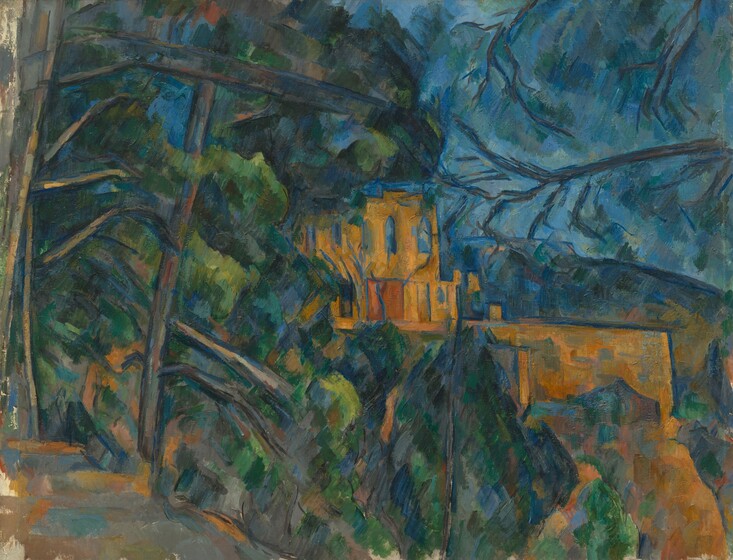The image depicts an intricate oil painting of a two-story building nestled within a dense forest. The building is highlighted with warm, yellow hues, reminiscent of a Santa Fe style house, and features a prominent balcony. Surrounding the structure, the verdant greenery of evergreen trees adds depth to the scenery, with hints of dark green and rich brown branches threading through the composition. On the mountainous backdrop, peeking through the foliage, various shades of green play harmoniously, while light blue patches break through the otherwise dark sky, suggesting a landscape themed with Greek or Roman influences. The light in the painting casts an orange-yellow glow on the building's off-white surfaces, evoking the impression of an unseen fire, lending a dynamic and somewhat mysterious ambiance to the forested valley scene. The detailed brushwork and interplay of color make the scene come alive, capturing the thick, immersive presence of the forest and rugged terrain.